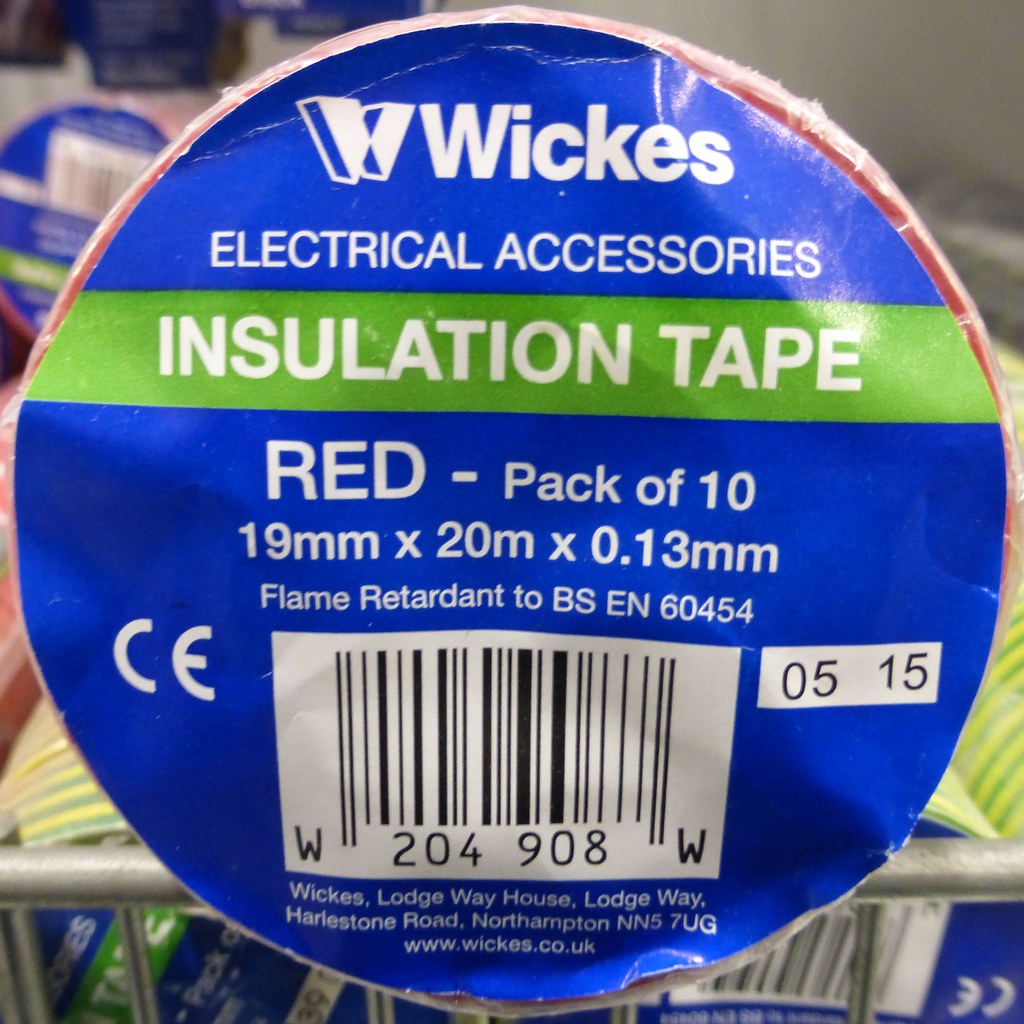The image depicts a close-up photograph of a circular roll of insulation tape packaging, likely taken in a hardware store. Dominating the picture is the round label of the tape, which occupies almost the entire image. At the top of the label is the brand name "WICKES" in white letters, accompanied by a stylized, three-dimensional "W" logo. Beneath this, the label reads "electrical accessories" in white text on a blue background. A green stripe follows, labeled "insulation tape." Below this stripe, additional product details are presented in white lettering, specifying a "pack of ten, 19mm x 20m x 0.13mm." To the left of the text, a white "CE" logo is visible, and to the right, there is a small white rectangle with the markings "05 15." At the bottom of the packaging, there's a large white rectangle containing a barcode and the company's address and website, "www.wickes.co.uk." The background behind the product is blurred, suggesting the setting is in a store.